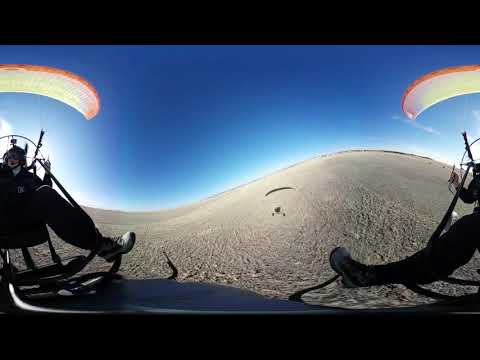The image captures two thrill-seekers engaging in hang gliding over a sandy, hilly landscape, likely a desert, with a fisheye lens distorting the scene and creating a unique perspective. The sky above transitions from a dark blue at the center to a hazy light blue and white towards the horizon. Each hang glider is located at the left and right edges of the image, partially cut off. The gliders feature orange canopies that form a U shape, blending yellow, white, and purple hues in the center. Both individuals are equipped with black helmets, black jumpsuits, white shoes, and are seated in their gliding apparatus with hands gripping the cables attached to their canopies. The person on the left, more illuminated by light, has their head visible, while the person on the right is mostly under shadow, with a noticeable foot sticking down. Below, the rippled, light gray sand shows faint foot impressions, and the shadows of the gliders stretch across the ground. The image, free of text, vividly conveys the adventure and excitement of hang gliding in a remote, sun-drenched terrain.